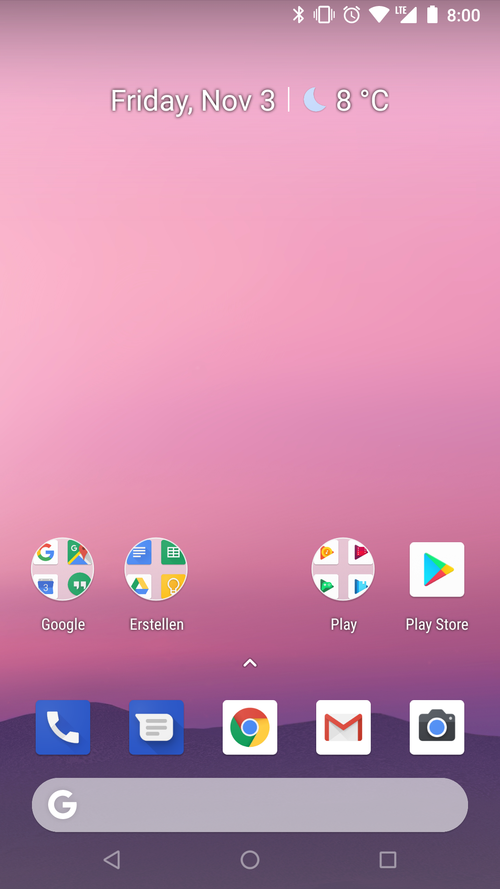This image showcases a cell phone screen with a vibrant purple background. In the top right corner, several icons are present, including the Bluetooth logo, an alarm clock, wireless signal strength, and cellular signal strength indicators, accompanied by the letters LTE. There's also a fully charged battery icon and the time displayed as 8:00. 

Just below these icons, the screen indicates the date, reading "Friday, November 3," next to a moon icon representing a waning crescent moon phase, with a temperature display of "8°C".

The central portion of the screen is dominated by the purple background, free from any text or icons, creating a substantial open space that draws the eye downward.

About two-thirds down, there is a cluster of icons within circular frames. The first circle includes the Google logo and white quotation marks, labeled "Google". Adjacent to it, another circle contains several icons, such as a blue square with horizontal lines, labeled "Earthstellen". On the right, a circular icon with four colorful play buttons in separate quadrants is labeled "Play". Following this, a square icon on the far right features the Google logo and is labeled "Play Store".

The bottom section of the screen has five square-shaped icons lined up: a telephone icon, a messaging icon, the Google Chrome logo, an envelope with an "M" on it representing Gmail, and a camera icon. Beneath this row of icons is a search bar, rounding out the user interface depicted in the image.